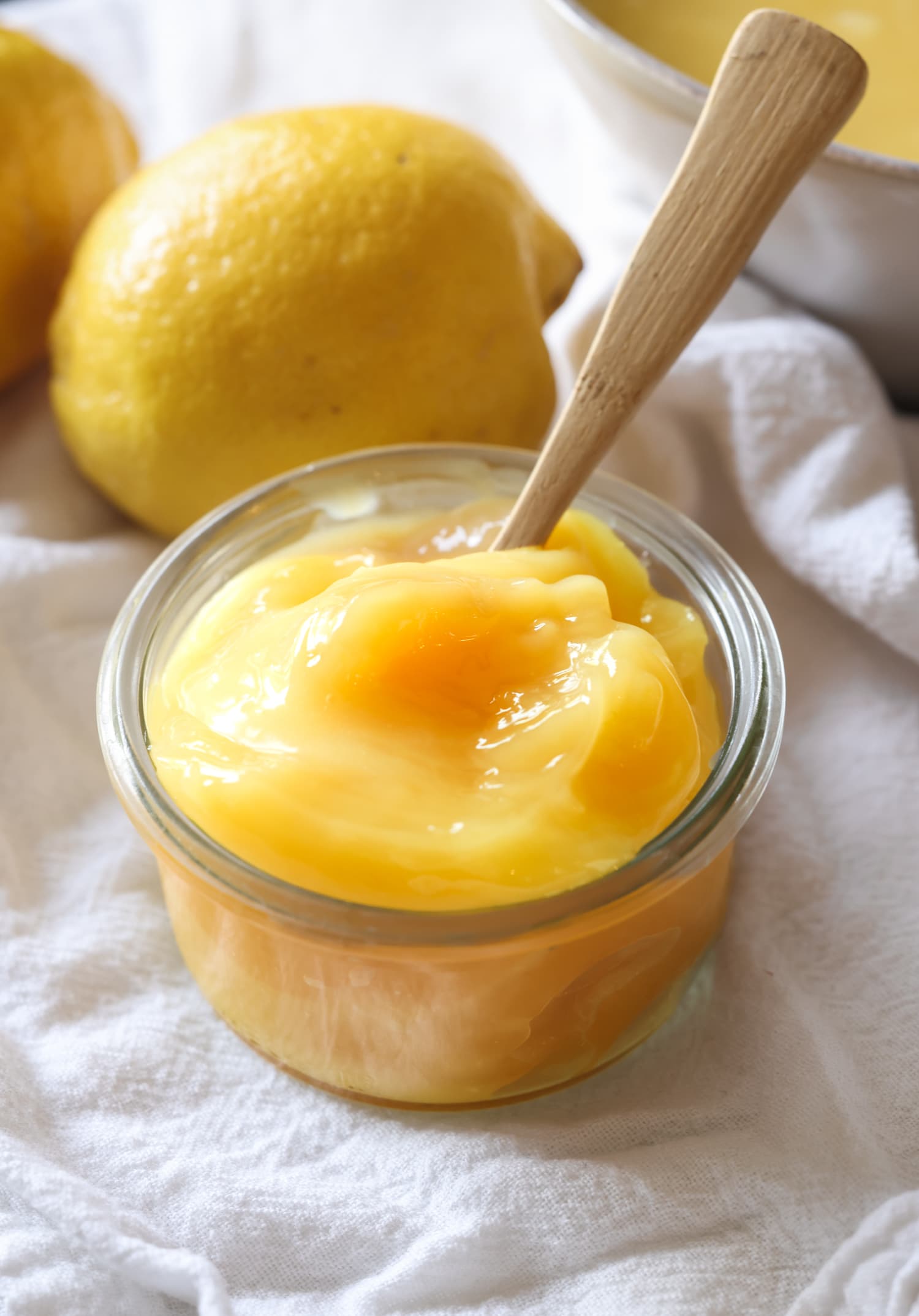This detailed photograph captures a delightful culinary scene, centered around a small glass jar filled with a thick, creamy yellow substance—possibly honey, whipped honey, lemon jelly, or a lemon custard. A light brown wooden spoon protrudes from the jar, adding a rustic touch. Positioned directly behind the jar are two vibrant yellow lemons, enhancing the fresh, zesty ambiance of the composition. To the upper right, partially visible, stands a larger white porcelain bowl containing a similar yellow mixture, suggesting that it might be related to or part of the same recipe. All these elements are arranged on a white, textured cloth that resembles a flower sack towel with noticeable ruffles and folds, creating a casual yet charming backdrop. The natural light streaming in, likely from a nearby window, elegantly illuminates the scene, making it look inviting and delicious.